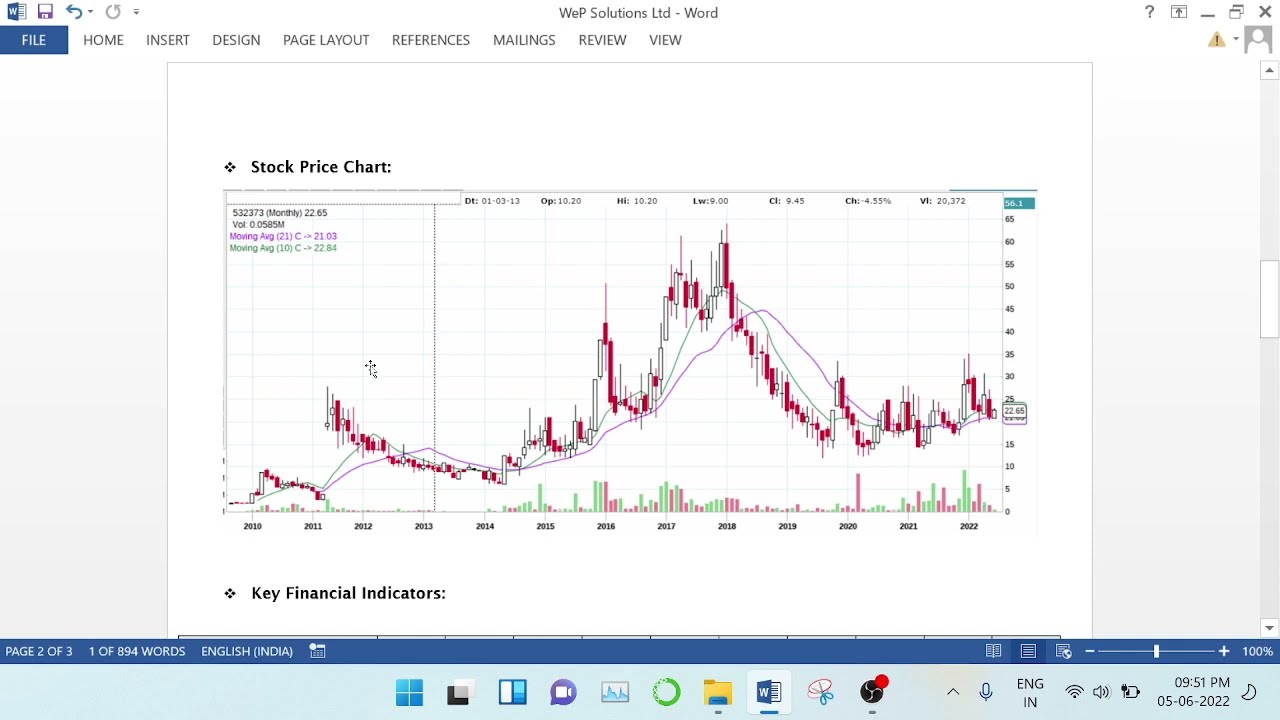This detailed screenshot showcases a Microsoft Word document titled "Web Solutions LTD Word" displayed on a computer screen. At the top of the screen, the typical Word menu tabs are visible: File, Home, Insert, Design, Page Layout, References, Mailings, Review, and View. The document contains a landscape-oriented, detailed "Stock Price Chart," featuring two prominent lines depicting the stock price trends over time, spanning from 2010 to 2023. Below the line graph, there is a bar chart component that provides additional data. The chart includes notations for Key Financial Indicators at the bottom, although full details require scrolling. The screenshot was taken on May 6th, 2022, at 9:51 PM, on a Windows machine in light mode, evidenced by the white toolbar at the bottom of the screen.